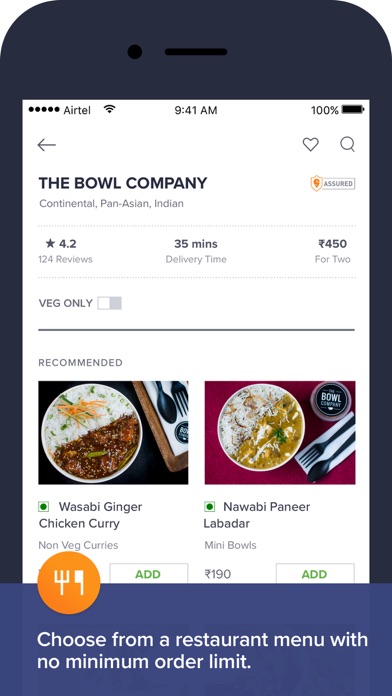The screenshot from a phone displays a user interface showcasing a food delivery application. The status bar shows the Airtel network, current time as 9:41 AM, and a full battery icon. The interface features several icons: a left-pointing arrow, a heart, and a magnifying glass. The header reads "The Bowl Company" with categories titled "Continental," "Pan-Asian," and "Indian," rated 4.2 stars based on 124 reviews. The estimated delivery time is 35 minutes and a meal for two is priced at $4.50.

A toggle switch labeled "VEG only" allows users to filter vegetarian options. Beneath this, a horizontal line separates the sections. The "Recommended" section displays two dishes. On the left is a plate with rice and brown beans accompanied by a silverware set wrapped in a napkin, labeled "Wasabi Ginger Chicken Curry" under the "non-veggie curries" category. To the right is a similar plate that appears lighter in color, labeled "Nawabi Paneer Labrador Mini Bowls." At the bottom of the screen, a note informs users that they can choose from the restaurant's menu with no minimum order requirement.